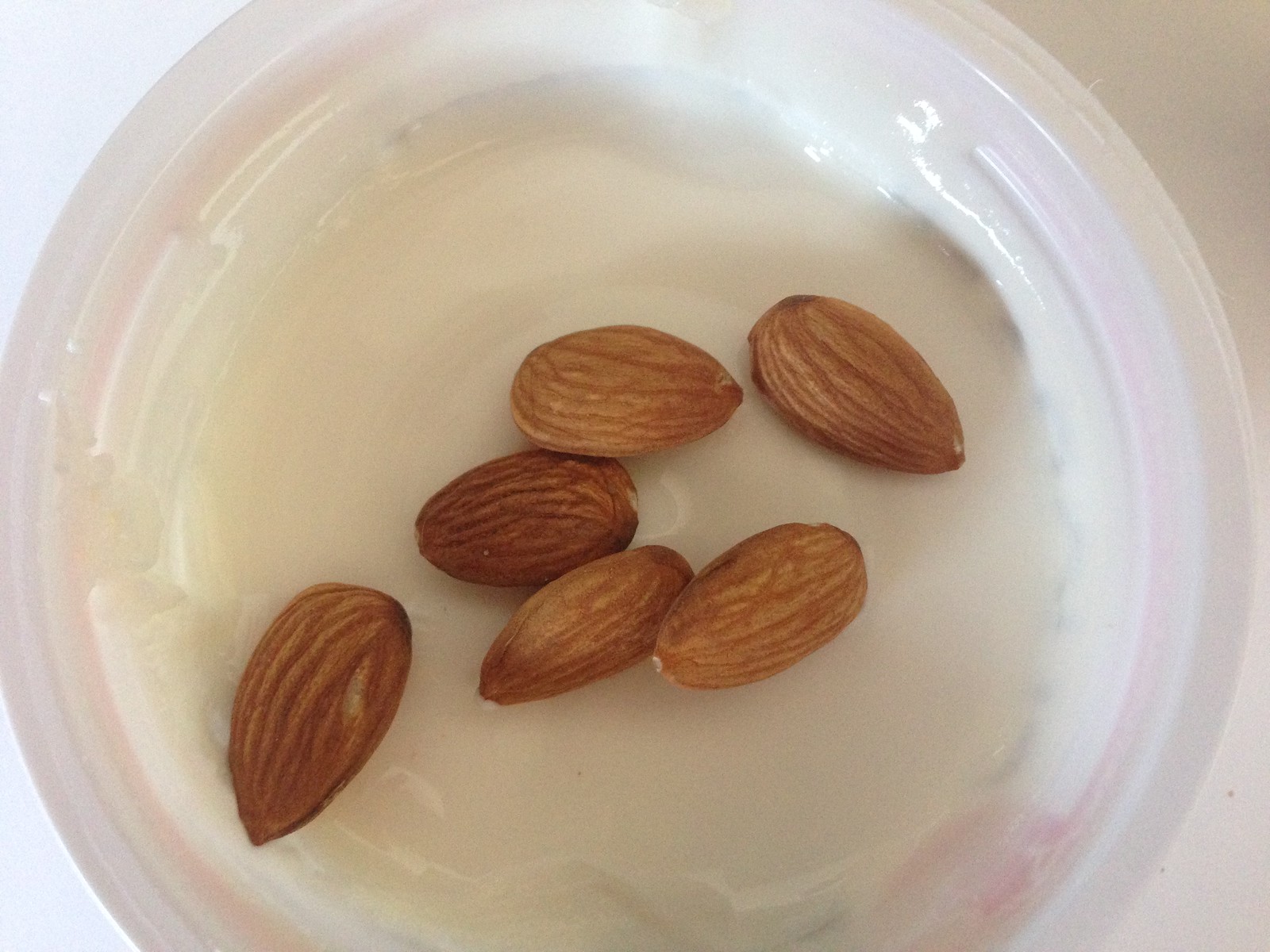This close-up color photograph captures an opened, round plastic container of pristine white yogurt, positioned on a neutral surface. The camera looks directly down into the container, showcasing six raw almonds meticulously arranged on the yogurt's smooth surface, which remains untouched and undisturbed. The container exhibits a faint pink ring around its rim, hinting at external packaging, and its circular shape occupies most of the frame, with some parts cut off at the top and bottom due to the zoom. The personal-sized yogurt pot acts as a subtle, creamy backdrop to the prominently featured almonds, enhancing their earthy tones and intricate details. The surrounding surface is a muted beige, blending seamlessly with the simple, yet elegant presentation of the yogurt and almonds.